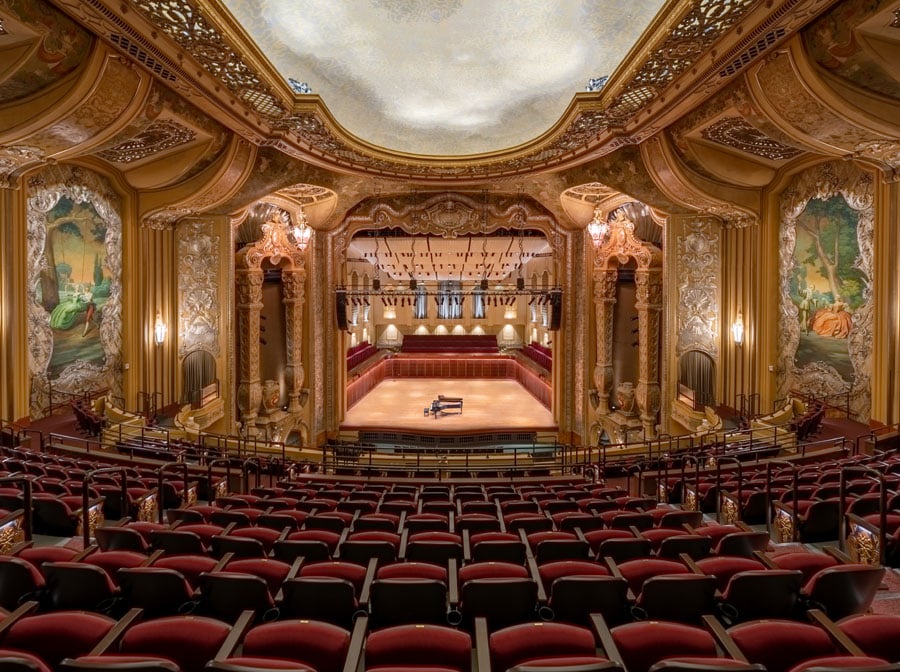This detailed photograph captures the opulence of a grand and beautifully ornate theater, taken from the back looking towards the stage. The auditorium features several rows of red seats and is adorned with intricately carved, sculptured wooden details and gold molding on the ceilings. The stage, situated at the far end, appears to house a small grand piano at its center, though it's faint in the distance. The walls are lined with individual picture slots containing artwork, adding to the theater’s majestic ambiance. The setting evokes the luxurious design elements reminiscent of historic, ornate Russian theaters. The lighting highlights the meticulous craftsmanship, suggesting excellent acoustics and an older architectural style, making the space both visually stunning and acoustically superior.